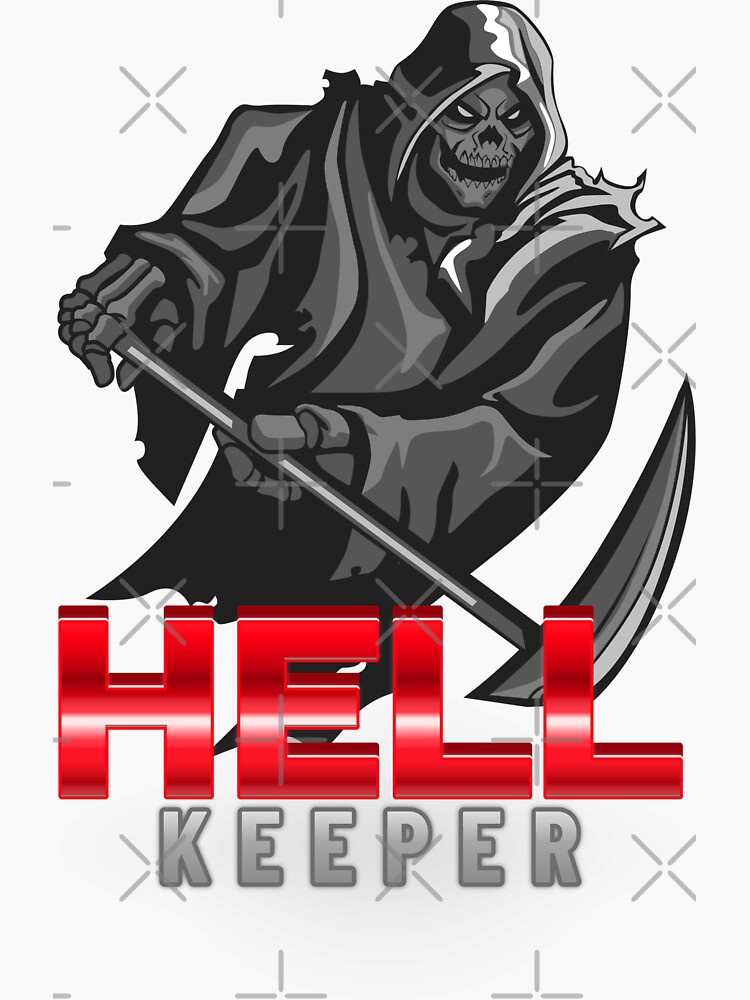This vertical, rectangular piece of computer art measures approximately five inches high and four inches wide. It features an off-white background adorned with alternating patterns of gray Xs and plus signs, resembling watermarks. Dominating the upper portion of the image, a dark gray depiction of the Grim Reaper is showcased. The Grim Reaper, with an angry skeletal face, is clothed in a long, black or dark gray robe with a hood, and is gripping a scythe angled toward the lower right. The bottom half of the image presents the bold, beveled text "HELL" in vibrant red, giving a 3D effect, followed by the word "KEEPER" in smaller, gray block letters with a dark gray outline. The overall composition is haunting and visually striking.